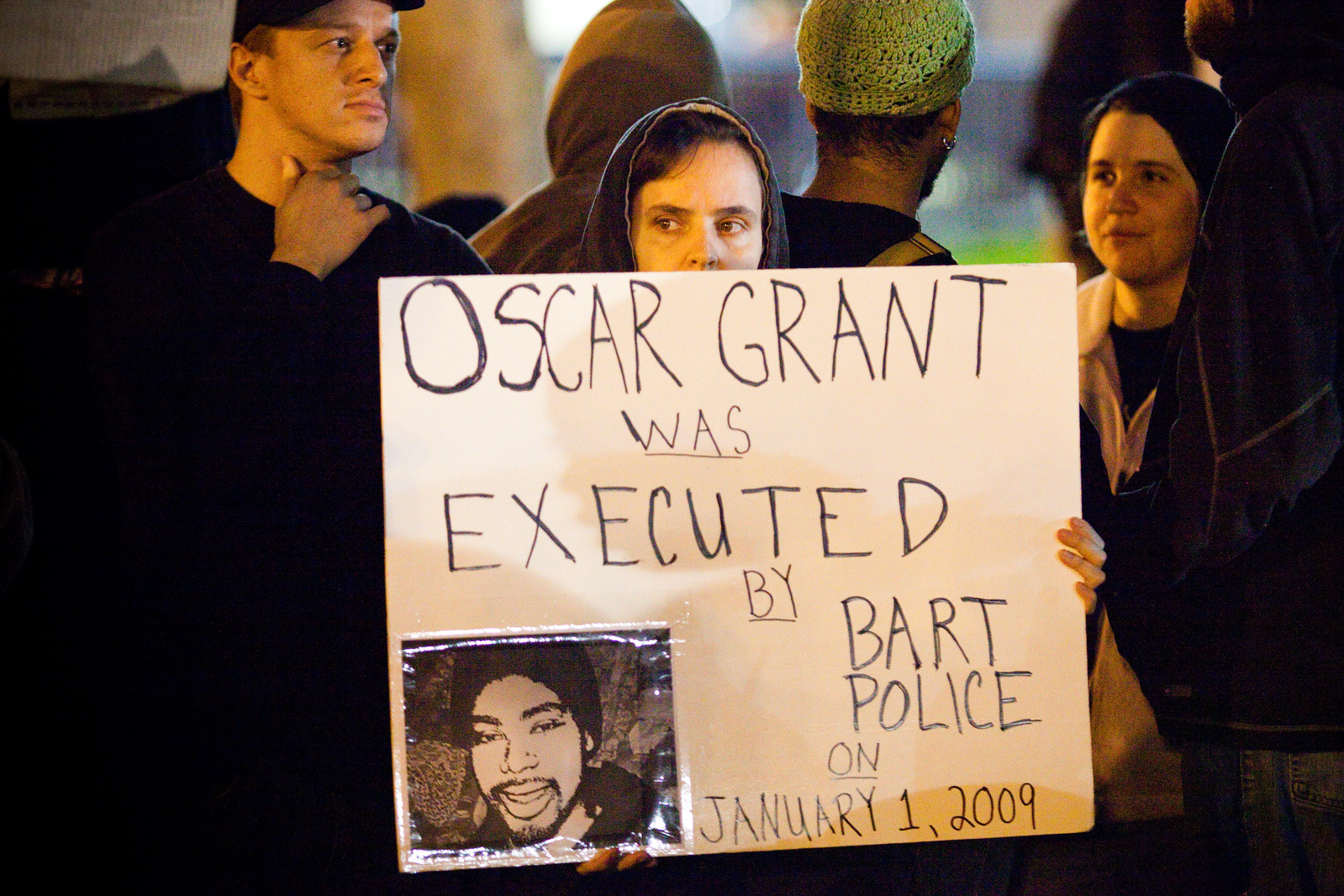In this image, a nighttime protest rally is depicted, focusing on a prominent handwritten sign centered in the frame. The sign, held by a woman whose face is partly visible from the nose up, reads in bold black letters on a white background: "Oscar Grant was executed by BART police on January 1, 2009." Below the text, on the lower left corner of the sign, is a black-and-white drawing of Oscar Grant, a black man with a mustache and wearing a cap. The woman's left fingers are seen gripping the sign as she stands amidst the crowd.

Around her, several other protesters are visible, most dressed in dark clothing. To the immediate top right of the sign, the head of a person with green hair is visible, while further to the left, the backs of two individuals can be seen—one wearing a hoodie and another also clad in dark attire. Another individual, identifiable by a green knit cap, faces away from the camera. In the backdrop, there is a combination of blue and green hues, blurred to keep the main focus on the protest sign and the partially visible crowd, highlighting the solemn atmosphere of the protest for Oscar Grant.